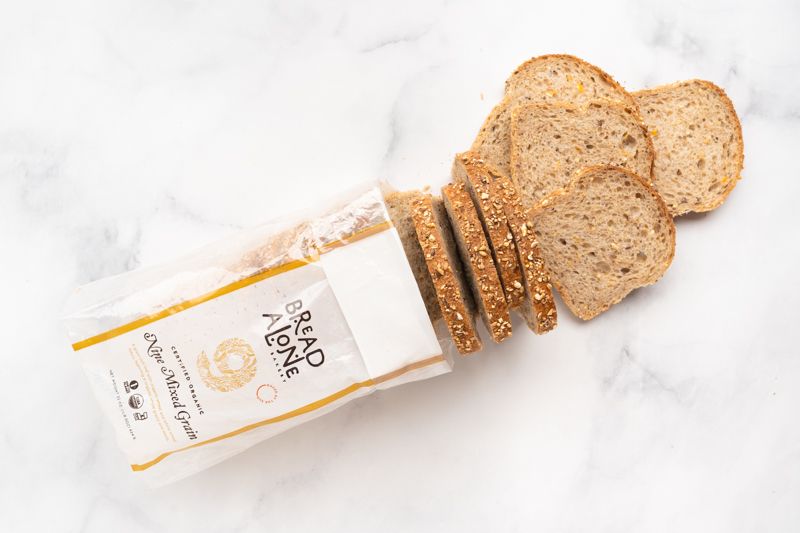The image depicts a partially opened loaf of bread on a white and faintly marbled countertop. The loaf, encased in a clear plastic package adorned with a white rectangular label featuring gold accents, bears the brand name "Bread Alone" in dark text. Prominently displayed on the bag is a grain-textured digit '9' with the description "Nine Mixed Grains" beneath it in black text. Part of the loaf, consisting of the last four slices, lies face-up just outside the opening of the bag. In addition, four more slices are standing upright beside these, showcasing the grainy surface of the bread. The remaining bulk of the loaf still sits within the clear package, giving the impression that the bread has spilled partially out of the bag onto the marble slab.